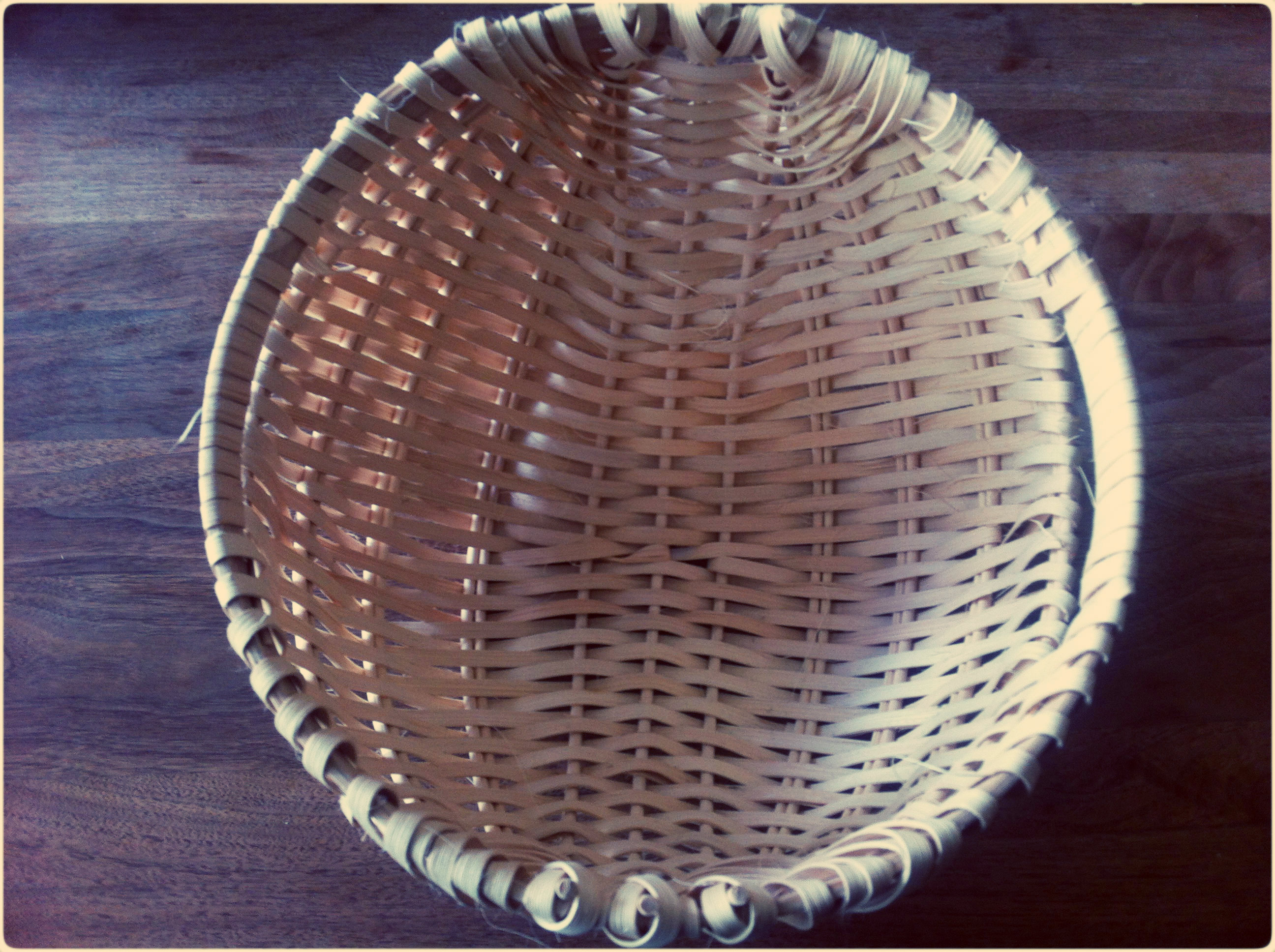This close-up photograph showcases a professionally woven, round wicker basket placed on a dark hardwood surface. The basket, primarily light tan in color, has an intricately woven design with a larger wooden band around the top and evenly spaced wicker strips forming its structure. The right side of the basket is illuminated, causing a creamy hue, while the center and left side remain in shadow, creating a gradient of color from light to dark. Although no handles are visible, there are indications of spaced weaving that may accommodate them. The wooden surface beneath, which could be a table or floor, features rich horizontal grains ranging from gray-brown to mahogany-brown. The surface also has a textured appearance with potential dust marks. The light, presumably natural sunlight, enters from the left, enhancing the detailed textures and shadows, making the basket the focal point of the image.